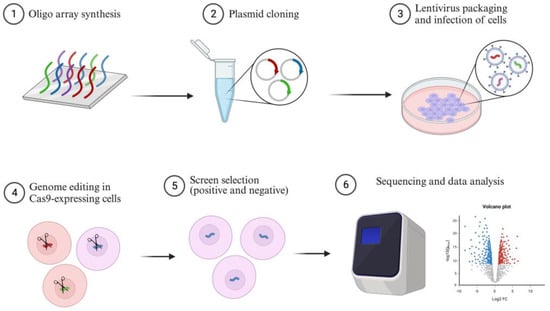The image illustrates a detailed six-step scientific process for genetic sequencing and DNA manipulation. Step 1, labeled "LIGO array synthesis," features a flat panel displaying multi-colored squiggly lines, symbolizing synthesized cells. These synthesized cells are then transferred to a test tube. In Step 2, "plasmid cloning" is depicted, where the cloned DNA material appears in a diagram showing a process with bottles and arrows in various colors (red, blue, and green). 

Next, in Step 3, the process of "lentivirus packaging and infection of cells" is shown with a Petri dish containing infected cells. Step 4 moves to "genome editing in Cas9 expressing cells," illustrated with scissors over the cells, highlighting the CRISPR-Cas9 technology for precise DNA editing. 

Step 5 involves "screen selection" where cells are sorted into positive and negative categories, depicted with squiggly lines inside the cells. Finally, Step 6, "sequencing and data analysis," is represented by a computer with charts and analytical data, indicating the culmination of the genetic sequencing and analysis process. This comprehensive diagram provides a step-by-step visual guide of the intricate procedures involved in genetic sequencing and DNA manipulation.